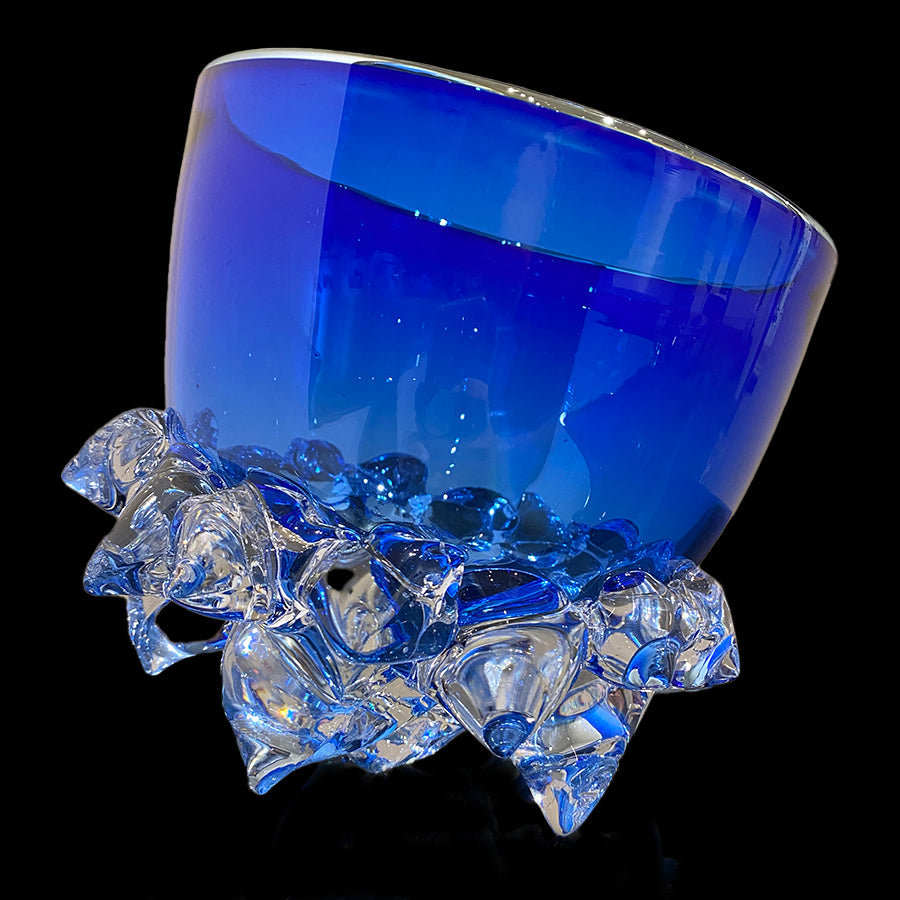Against a solid black background, a stunning crystal glass commands the center of the image. The glass, short and round in shape, exudes a vibrant blue hue that shimmers with the light. The base of the glass is adorned with intricate, ice-crystal-like protrusions fused to the main body, giving an impression of frozen spikes bursting outward. These embellishments are transparent with a hint of blue, reflecting the light and casting a beautiful, glistening effect. The rim of the glass catches the light in a way that creates a silvery glow. This artistic piece, possibly a vase or an ornate cup, appears empty, allowing the viewers to appreciate the intricate design and captivating colors highlighted by the carefully placed lighting.